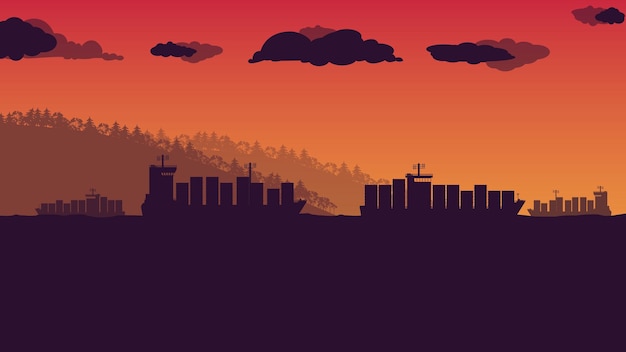This detailed, horizontal image appears to be a minimalist, graphic representation of a side-scrolling game or digital artwork. Dominated by a vibrant, moody palette of oranges, browns, and blacks, the scene features the silhouettes of four cargo ships, laden with shipping containers. Two of these ships occupy the foreground, while two more appear farther in the distance, rendered in lighter shades. The lower third of the image is a solid black, evoking the impression of an ocean or large body of water. The upper two-thirds is a striking depiction of an orange sky, transitioning from lighter tones near the horizon to darker hues at the top, punctuated by dark brown and black clouds. Conifer-clad mountains emerge from the left, descending towards the right in a faded, misty silhouette, enhancing the layered depth of the scene. The overall atmosphere is one of serene desolation, underscored by the absence of any human figures.